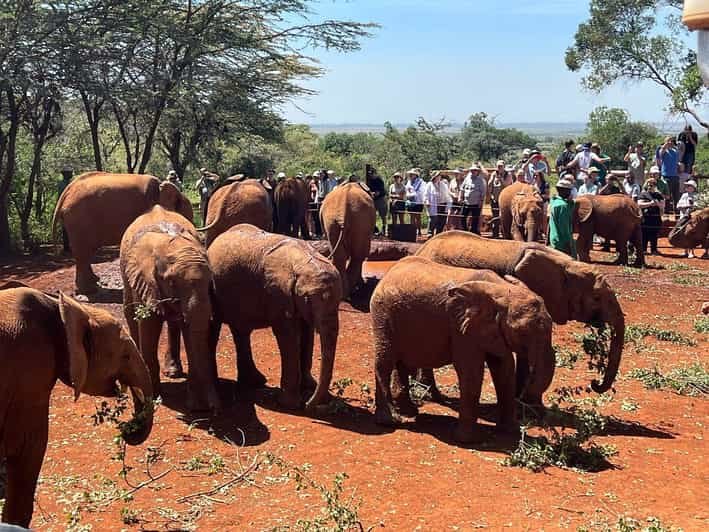This vivid photograph captures a bustling scene of at least a dozen elephants, the majority of which are endearing, small baby elephants, set against a backdrop of red-brown soil. The elephants' skin, tinged with the reddish hue of the dirt, suggests they've been dusting themselves. Scattered around the enclosure are green branches and leaves, which the elephants are eagerly munching on, adding to the lively atmosphere. The setting appears to be an elephant sanctuary or similar enclosure, surrounded by a mix of trees and a gated boundary. The clear blue sky suggests a bright, sunny day, casting sharp shadows across the scene. In the background, tourists, many wearing hats and snapping pictures, observe the elephants with fascination. The juxtaposition of the small elephants against the taller human spectators, particularly noticeable in the top right of the image, emphasizes the youth and delicacy of these majestic creatures.